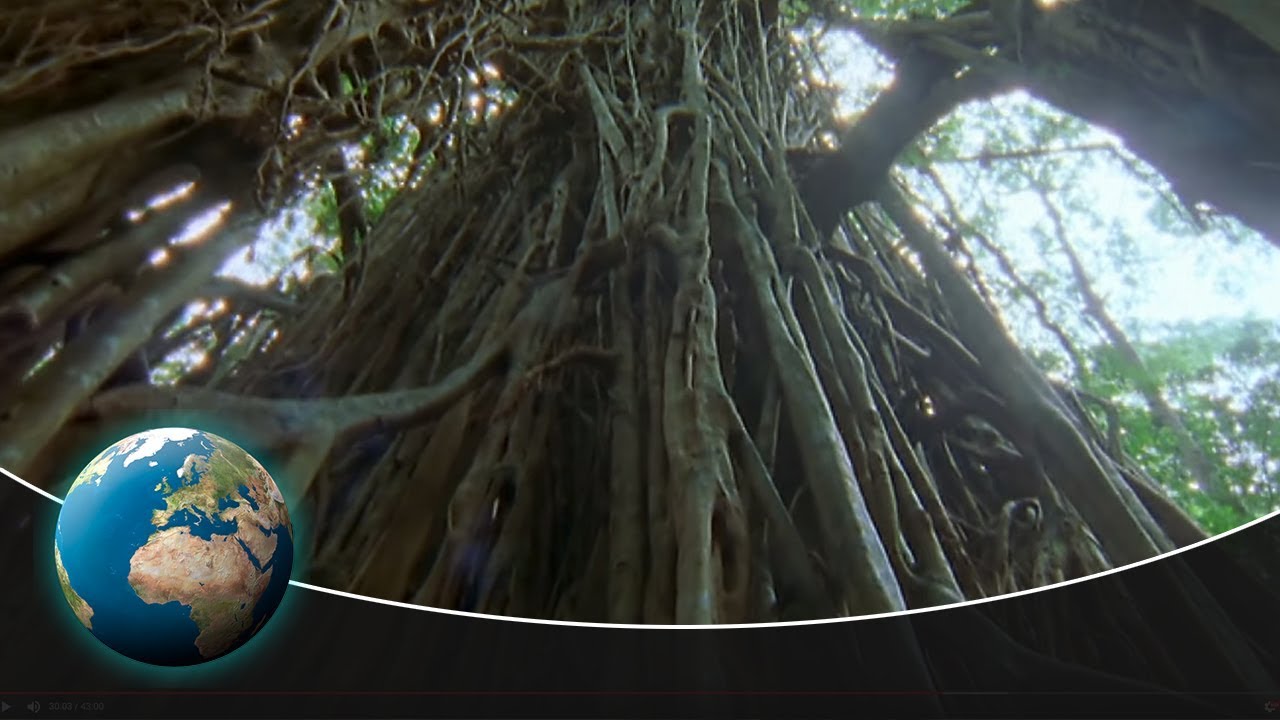The image appears to be a slightly lower-resolution photograph taken outdoors, possibly in a tropical rainforest or jungle. The viewpoint is from below, looking up at an old tree or tangled mass of roots and branches, which are interwoven and covered in vines. The sky is clear and blue, with the sun shining brightly, illuminating the scene. In the bottom left corner, there is an inset image of a globe, showing Africa and parts of Europe, possibly highlighting the geographical focus of the context, which might be a documentary or part of a study on the environment. The photograph's edges are bordered by a white band, adding a framed look to the image. The background features lush greenery with thin trees and abundant leaves.